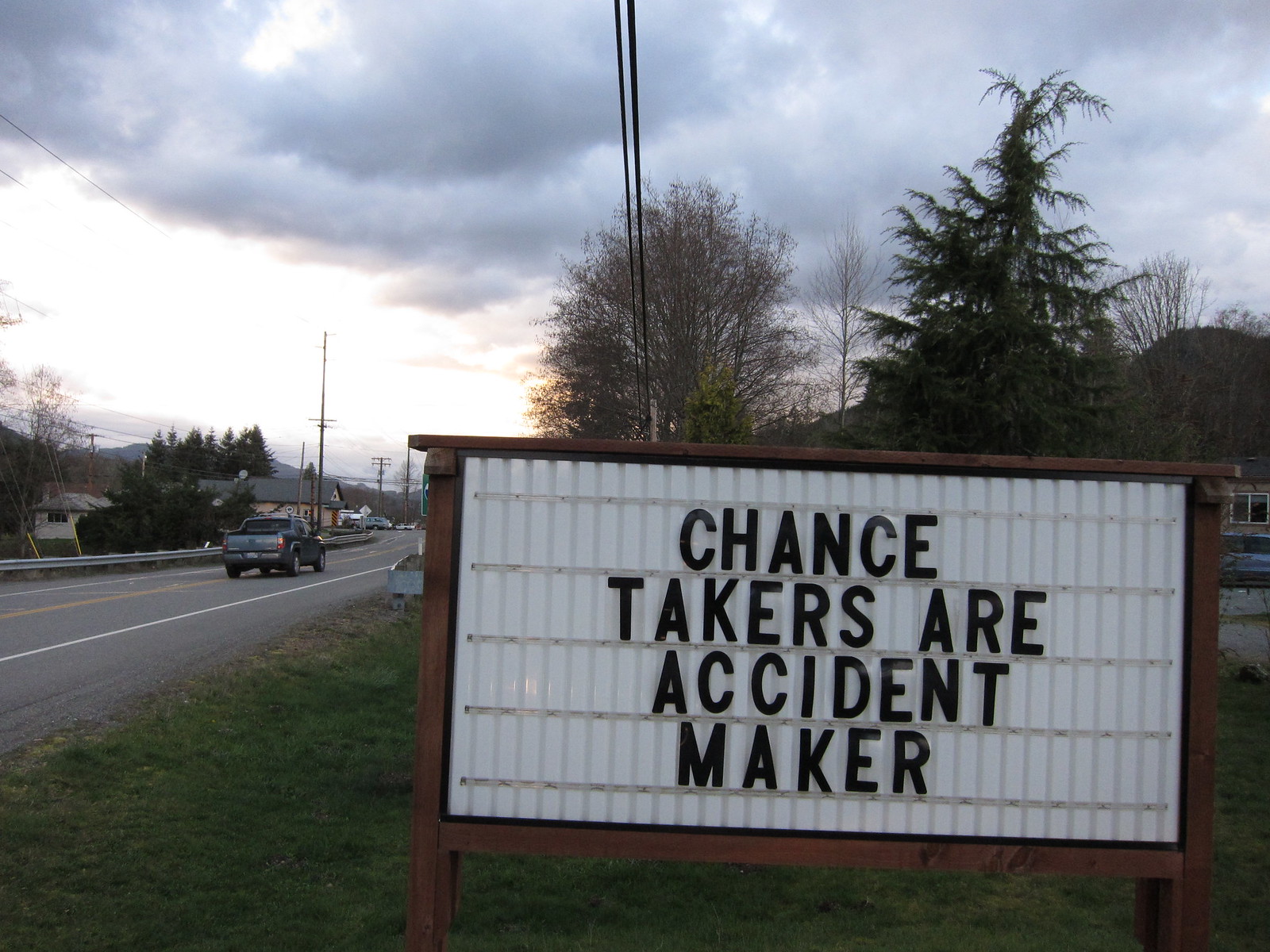A detailed description of the image shows a rectangular sign prominently displayed in a grassy yard. The sign, framed by wooden posts and border, features white panels with black lettering that reads: "Chance takers are accident maker," with a missing 's' on "makers." The yard is adjacent to a road on the left, where a truck is seen driving by. In the background, there is a building, possibly a community center or office, with a shed situated to the left of it. A cluster of trees with dark green foliage creates a natural backdrop for the scene. The sky occupies the upper half of the image, appearing bright white with patches of light gray clouds. To the right, two trees stand distinctly—one sparsely leafed and the other lush with dark green leaves. The overall setting exudes a calm, ordinary day in a suburban or rural area.